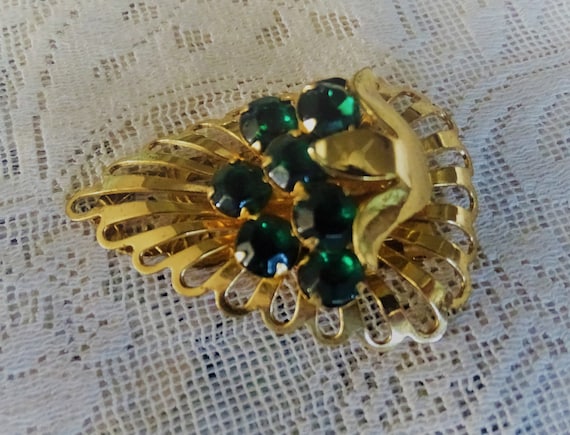This staged, full-color square photograph captures an elegant piece of jewelry—possibly an earring or brooch—set against a white doily backdrop. The jewelry features a gold, shield-like design composed of concentric loops. At its heart are seven round green gemstones, which could be emeralds, although they lack the sparkle typically associated with diamonds. The overall shape of the piece is somewhat triangular, with rounded sides and possibly pointing to the left. The central gemstone arrangement may resemble a bunch of grapes, surrounded by what appear to be three gold leaves, all meticulously crafted from elongated gold loops. The photograph is lit with artificial lighting, emphasizing the intricate details of the jewelry and the texture of the white crocheted or embroidered cloth beneath it.